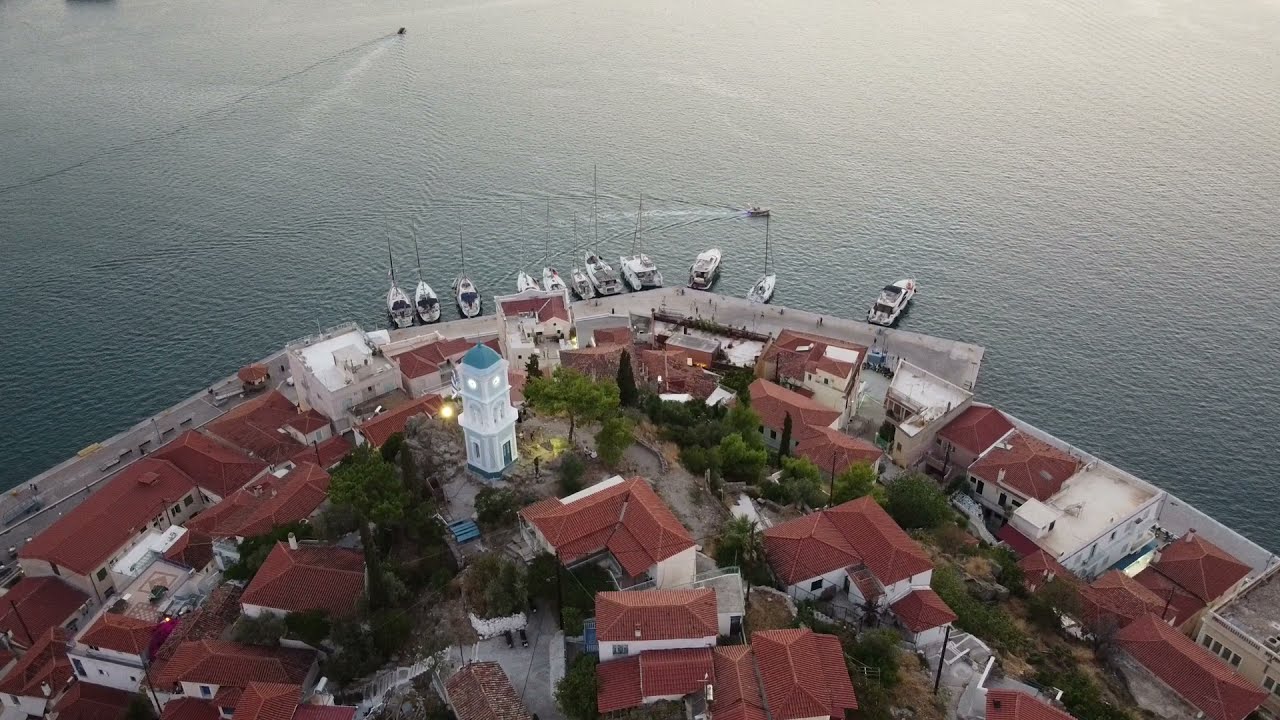This aerial image depicts a picturesque dockside village characterized by uniformly white buildings adorned with warm brown, or red-tiled, roofs. Nestled among these buildings are lush green trees that add to the village's charm. A prominent feature is a taller white building near the mid-left, distinguished by its blue rounded roof, possibly a church, complete with a clock and illuminated dome. This edifice stands about three stories tall. The scene is vibrant yet serene, with the village occupying one-half of the image while the other half is dominated by a calm, rippling body of water. The water hosts about ten sailboats docked along a concrete pier that gently curves in a horseshoe shape around the village. The overall layout of the land is somewhat rounded, enhancing the sense of a snug, well-protected harbor town.